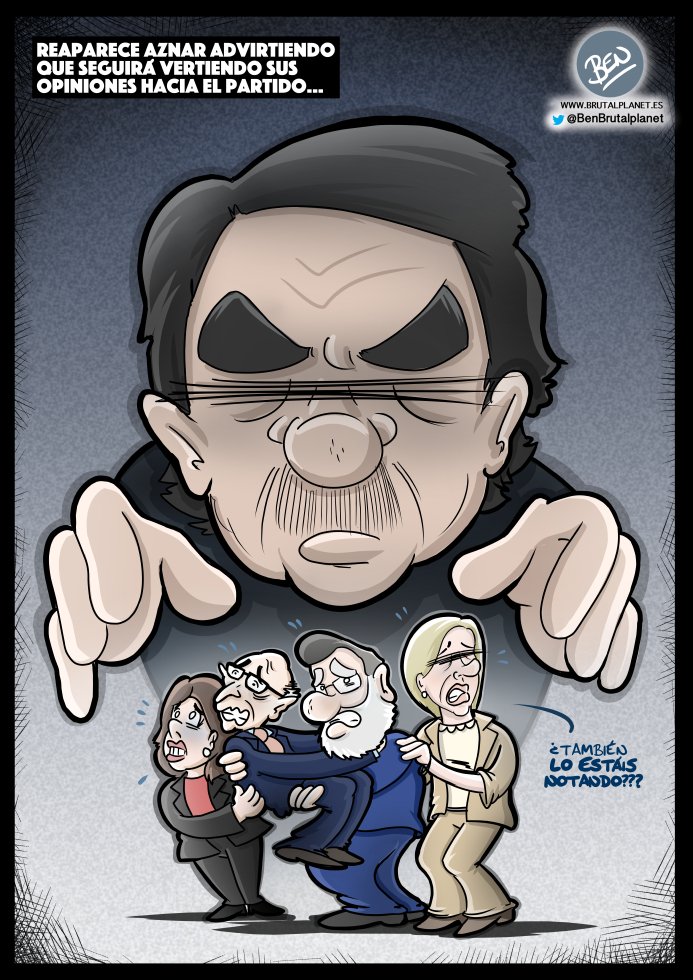The detailed political cartoon, rendered in Spanish, depicts an ominously large man with black hair, black eyes, and a mustache, designed with cat-like features, exuding evil. This central figure, shrouded in black and gray, ominously hovers over a group of four smaller, terrified individuals positioned between his outstretched, grasping hands. The image vividly portrays these unfortunate people, dressed in various colored suits—gray, blue, and beige—who appear as though they are about to be captured. Among them, one person clutches another protectively in their arms, representing apparent desperation and fear. Handwritten Spanish text adorns the top left, bottom, and right-hand corners of the cartoon, albeit in script difficult to decipher due to its small size. The dark tones and menacing posture of the large man amplify the terror of the smaller figures, encapsulating the oppressive and predatory dynamic conveyed by the artist.